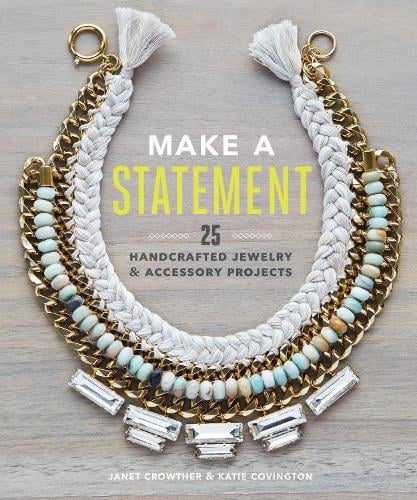The advertisement showcases a meticulously designed necklace against a light beige-gray, wood-textured background. The centerpiece necklace, forming a U-shape around the central text, features a braided rope in the inner layer, flanked by rows of gold and a striking combination of turquoise and off-white beads. At the base, five rectangular stones add a touch of elegance. Boldly placed in the center, white and yellow fonts proclaim "make a statement," followed by "25 handcrafted jewelry and accessory projects" in black font. The designers, Janet Crowther and Katie Covington, are credited at the bottom in white text, emphasizing the ornate and sophisticated nature of their handcrafted creations.